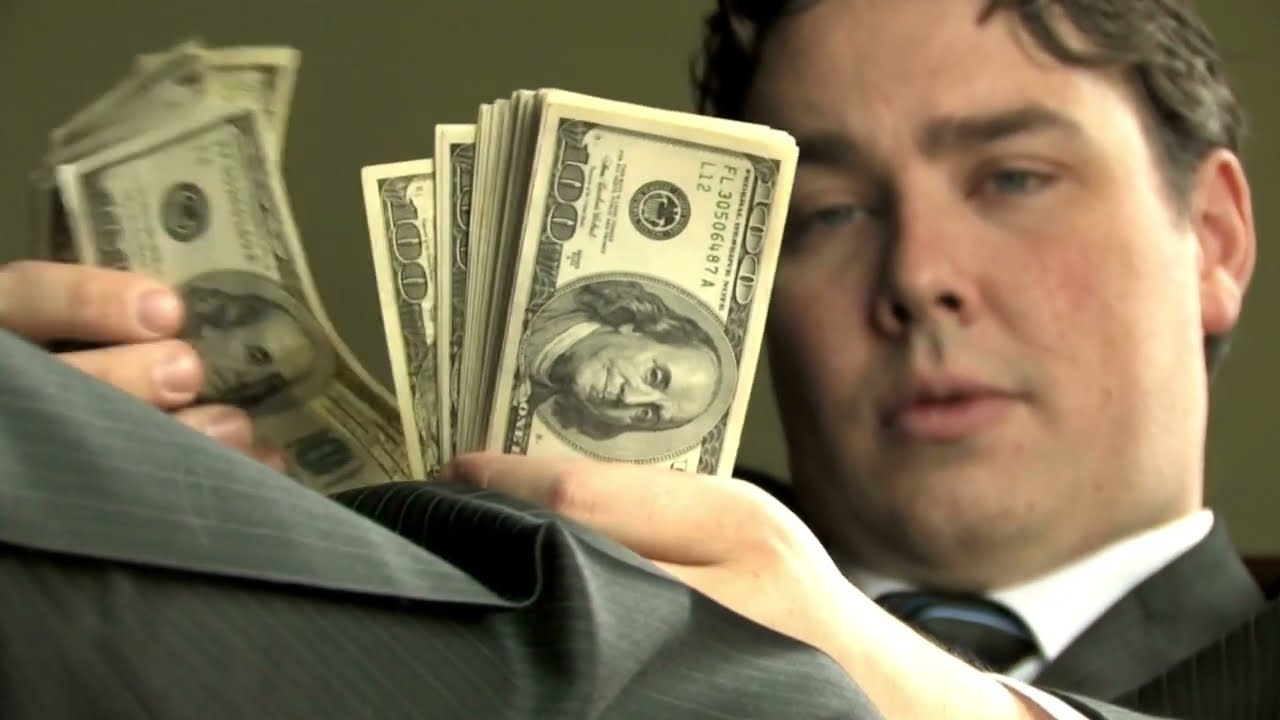In this wide rectangular image, a man is prominently featured against a dark green wall background. His face occupies the entire right side of the frame, displaying short brown hair, blue eyes, and an inquisitive expression with slightly parted lips. He is dressed in a white collared shirt paired with a black and blue striped tie, under a gray pinstripe suit with only a portion of it visible. The visible part of his suit extends to the left corner of the image, where his hands, holding stacks of $100 bills, rest. His right hand grips a thick pile of the bills while his left hand holds a few, suggesting he might be in the process of counting them. The man appears serious and focused as he attends to the substantial amounts of money he holds.